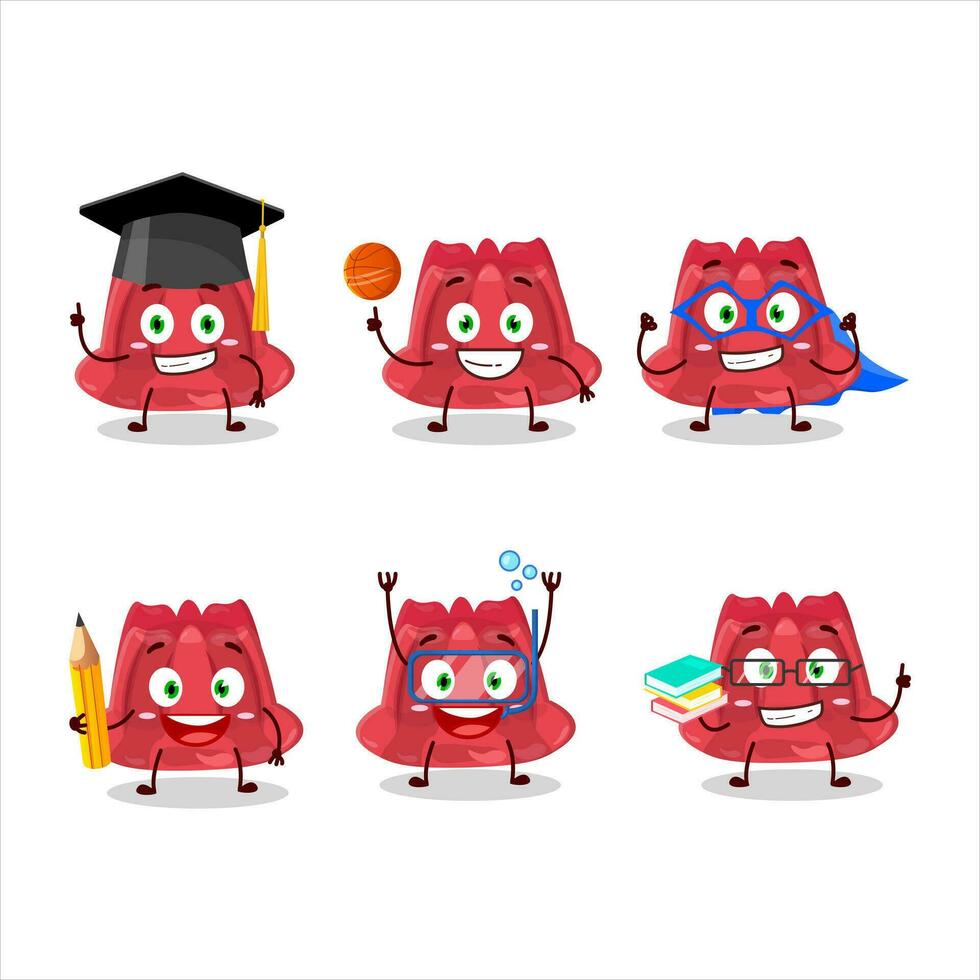The image depicts six cartoonish, red, strawberry jello characters, each with a face, stick arms, and legs, arranged in two rows of three. Each jello character embodies a unique role or occupation. Starting from the top left, the first jello wears a graduation cap with a tassel, raises its right arm with a thumbs-up gesture, and displays a small smile, characterized by its green eyes. To its right, the second jello balances a spinning basketball on its right finger, featuring a wide grin. The third jello on the top row masquerades as a superhero, donning a blue domino mask and an electric blue cape, with both arms raised in a victorious pose.

Moving to the bottom row, the first jello on the left holds a yellow pencil, showcasing a wide-mouthed smile. Next to it, the middle jello appears underwater, equipped with a blue scuba diving mask and surrounded by bubbles, arms lifted in an excited gesture. The last jello on the bottom right wears pince-nez style glasses and holds a stack of three books—green, yellow, and red—while raising its left thumb, giving a scholarly impression with its green eyes. All jellos have a distinct bell-shaped body with a ridged top, small black hands, and feet.